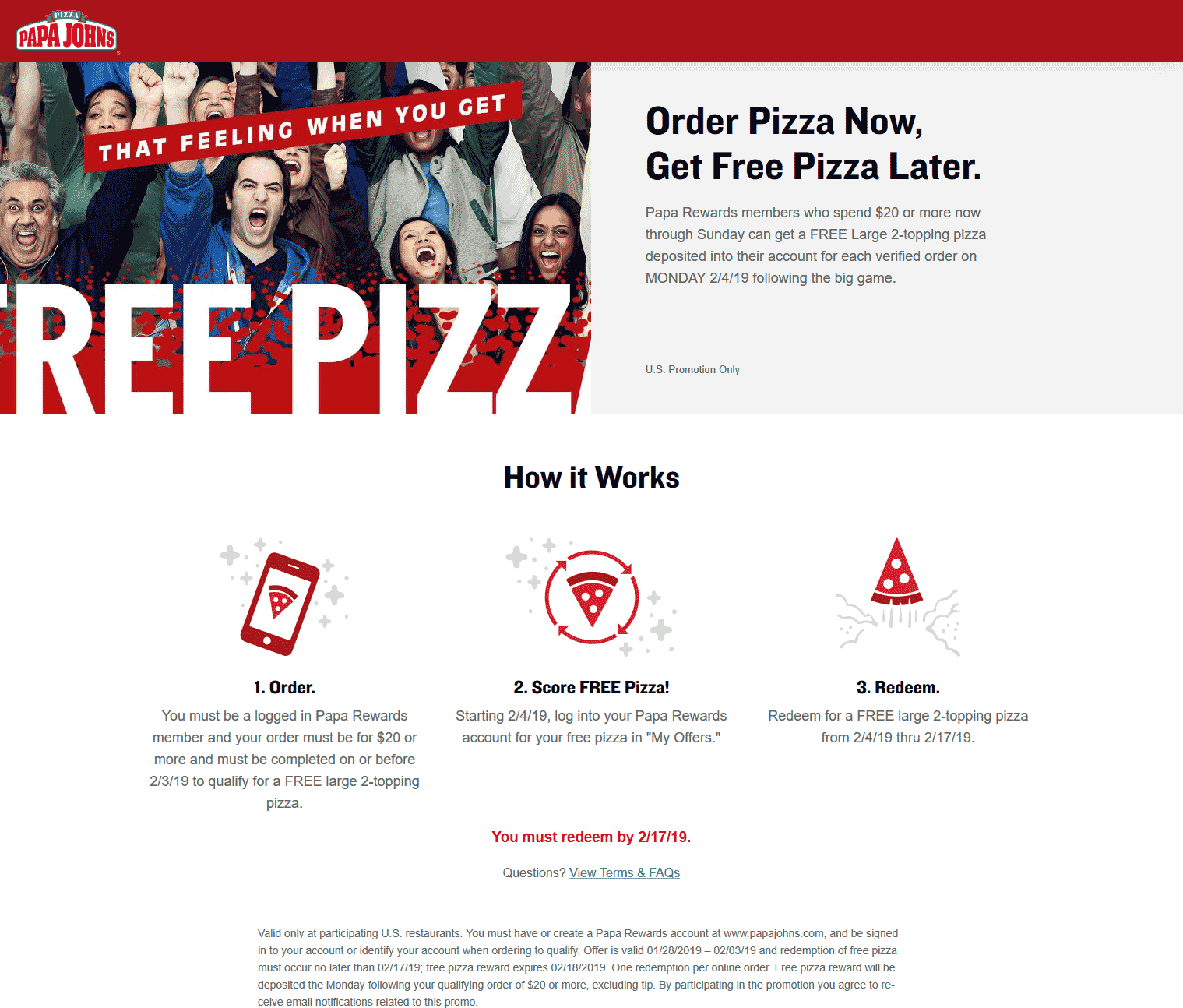The image from Papa John's displays an energetic celebration with several people raising their hands in excitement. A vibrant ribbon graphic spans across the top, emblazoned with the phrase "That feeling when you get" in bold letters. However, due to the image cropping, only "R-E-E-P-I-Z-Z" is visible, hinting that the phrase should read "free pizza" in large, capital letters below. The lower part of the image includes a step-by-step guide on how to earn free pizza: 

1. **Order Pizza Now** - illustrated with an icon of a smartphone displaying a slice of pizza.
2. **Score Free Pizza** - indicates that each order brings you closer to a reward.
3. **Redeem Free Pizza** - emphasizes that after accumulative purchases, you can enjoy free pizza.

The overall message highlights that the more pizzas you purchase, the quicker you'll earn free pizzas from Papa John's.